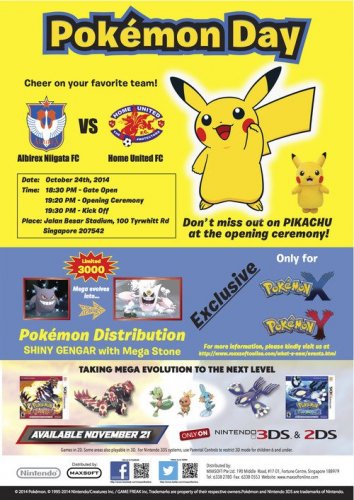This vibrant advertisement promotes an exciting Pokémon Day event. At the top, bold yellow letters with black and blue borders announce "Pokémon Day" against a yellow background. Just beneath this, the text "Cheer on Your Favorite Team" invites fans to join in the excitement. 

The central section of the ad features a matchup between two icons: a mostly blue icon representing Albirex Niigata FC on the left, and a mostly red icon for Home United FC on the right. It indicates a face-off between the two teams.

Below this, within a neatly organized box, essential event details are provided:
- **Date:** October 24, 2014
- **Times:**
  - Gates open: [time not specified]
  - Opening Ceremony: [time not specified]
  - Kickoff: [time not specified]
- **Venue:** Jalan Besar Stadium, 100 Tyrwhitt Road, Singapore

Adjacent to these details, a cheerful Pikachu is depicted, smiling and waving at viewers. To the right, a smaller, shocked Pikachu is shown with the text, "Don't miss out on Pikachu at the Opening Ceremony."

The bottom section of the advertisement highlights a special Pokémon distribution:
- **Offer:** Shiny Gengar with Megastone
- **Exclusivity:** Only for Pokémon X and Pokémon Y
- **Availability Date:** November 21

Several elements, including colorful graphics and Pikachu artwork, make this a noteworthy and engaging announcement for Pokémon enthusiasts.